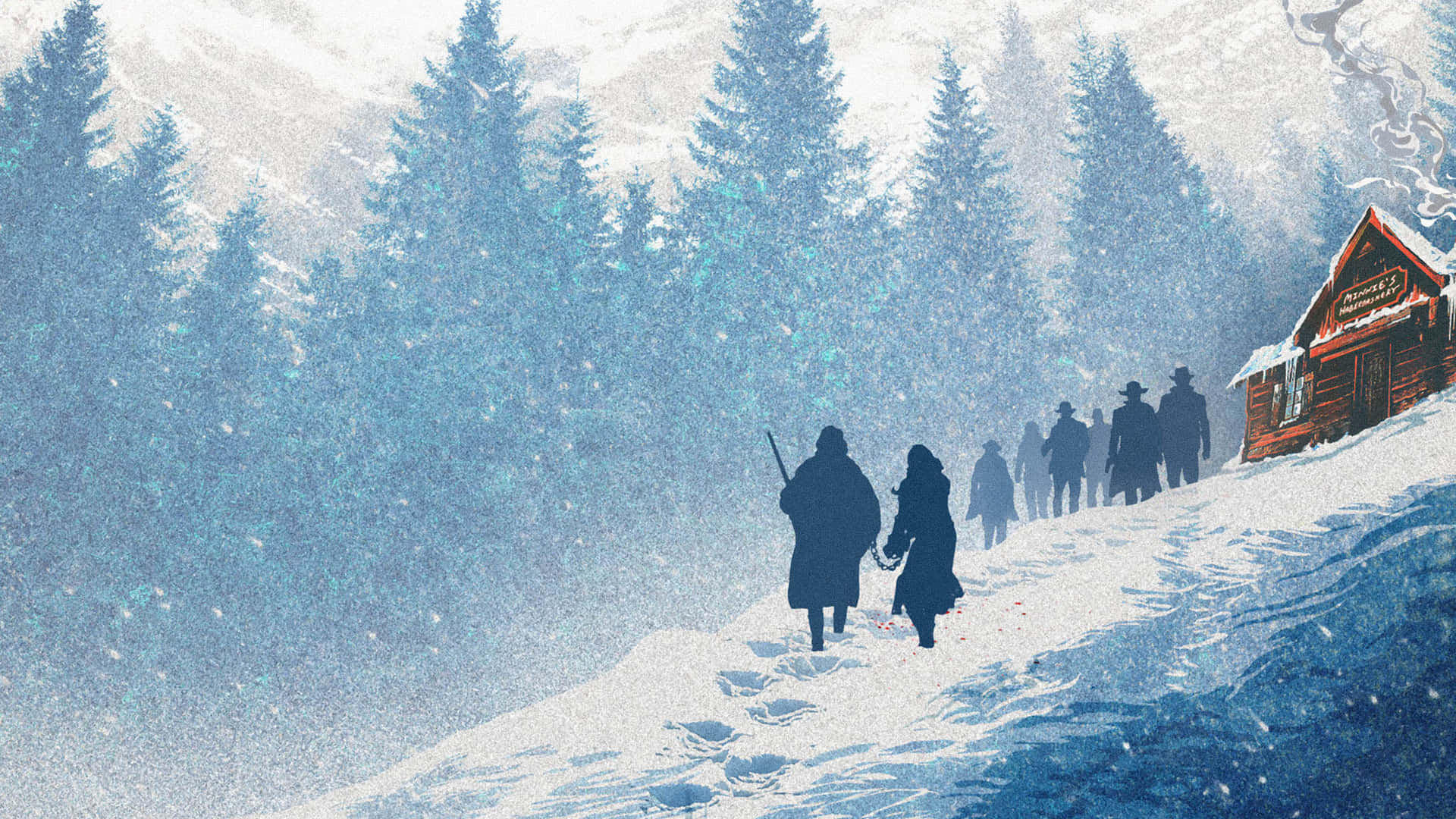In this oil or acrylic painting, a group of silhouetted people traverse a snowy mountainside towards a rustic log cabin. The scene is enveloped in a heavy snowfall, which mutes the surrounding evergreens into a misty backdrop. The dark silhouettes of the men, most adorning hats that resemble top hats or western style, walk in a line up the slope, leaving visible tracks through the snow. At the forefront, a man with a rifle in his left hand pulls a woman by a chain, indicating she is a prisoner. The woman, possibly in a dress, follows reluctantly behind. Ahead, about seven or eight more silhouetted figures are discernible. The cabin, constructed with reddish-brown wood, possibly cedar, stands prominently near the top of the ridge. Icicles hang from its eaves, reinforcing the cold, wintry atmosphere. A large, unreadable sign hangs over the cabin's entrance, suggesting it might serve a business purpose. The entire scene captures a bleak, Wild West landscape, dominated by the stark contrasts of blues, blacks, and the white snow.